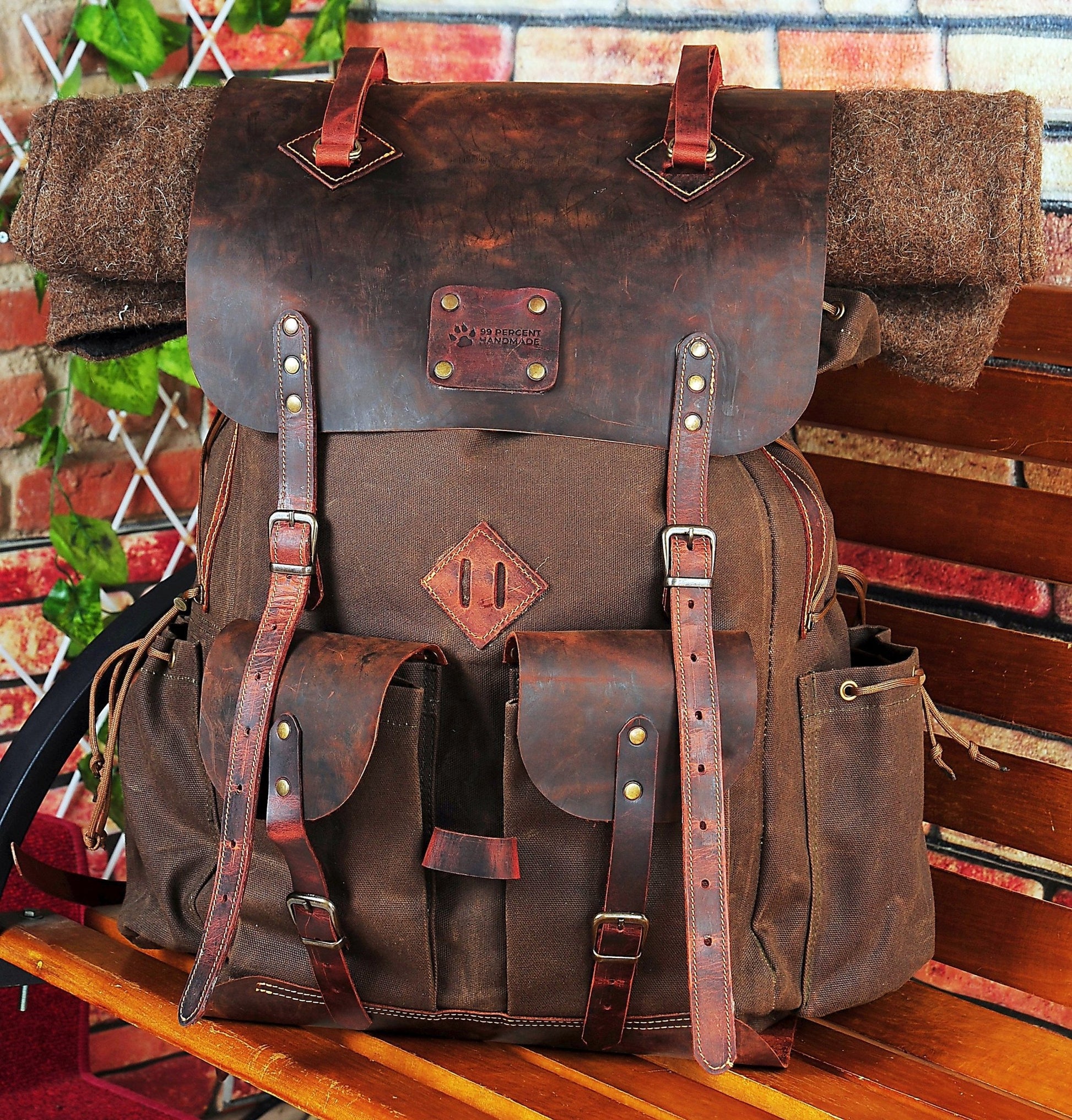A photograph shows a large, worn-out brown leather backpack placed on a shiny, warm brown wooden bench with black metal railings. The backpack, seemingly designed for hiking or outdoor use, features multiple compartments and straps: two leather belts securing the main large flap, two smaller front pockets with leather flaps, and two open side pockets with drawstring closures. Notably, there is a rough, woolen or burlap material rolled up and tucked under the top flap, stretching outwards from both sides. A bolted-on, small leather square patch near the top of the flap exhibits a paw print or bear print design, with unreadable text that hints at being 99% handmade. The backdrop includes a brick wall partially covered by a chain link fence and greenery with bright green leaves and weeds growing through, adding a touch of natural vibrancy to the scene.